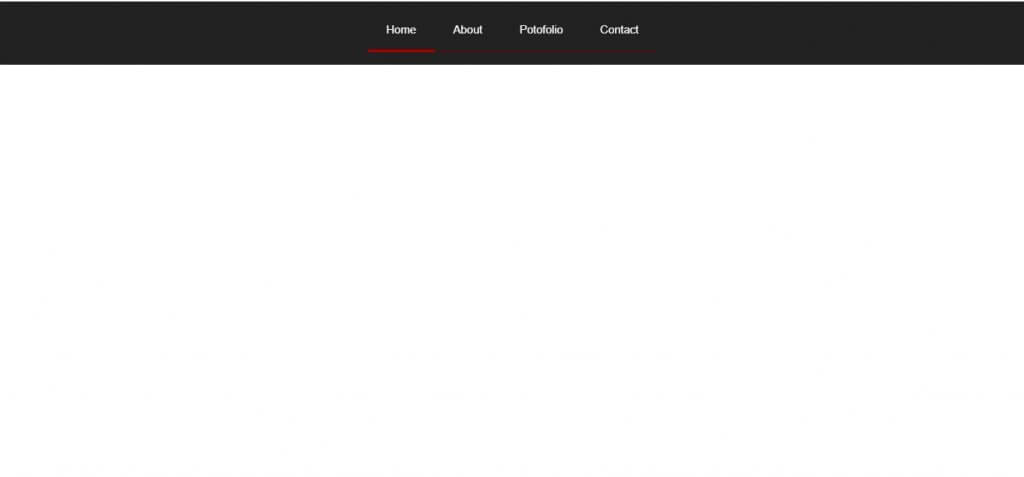The image depicts a minimalist web page interface. At first glance, it appears as if the page is slow to load, but it is fully loaded and just sparsely populated. The top part of the screen features a thin black horizontal navigation bar that lists four menu options: Home, About, Portfolio, and Contact. A red underline beneath the "Home" menu item indicates it is the selected page. The interface does not have any other visible elements or borders, blending seamlessly into the surrounding white background, which creates ambiguity about whether it is being viewed on a computer screen or another type of device. This design suggests the website could be related to home design, featuring visually appealing products or services, evidenced by the presence of a portfolio section where users can likely view examples of their work. While the clean and simple layout hints at a focus on aesthetic appeal, the homepage itself is notably sparse, potentially failing to immediately engage visitors.